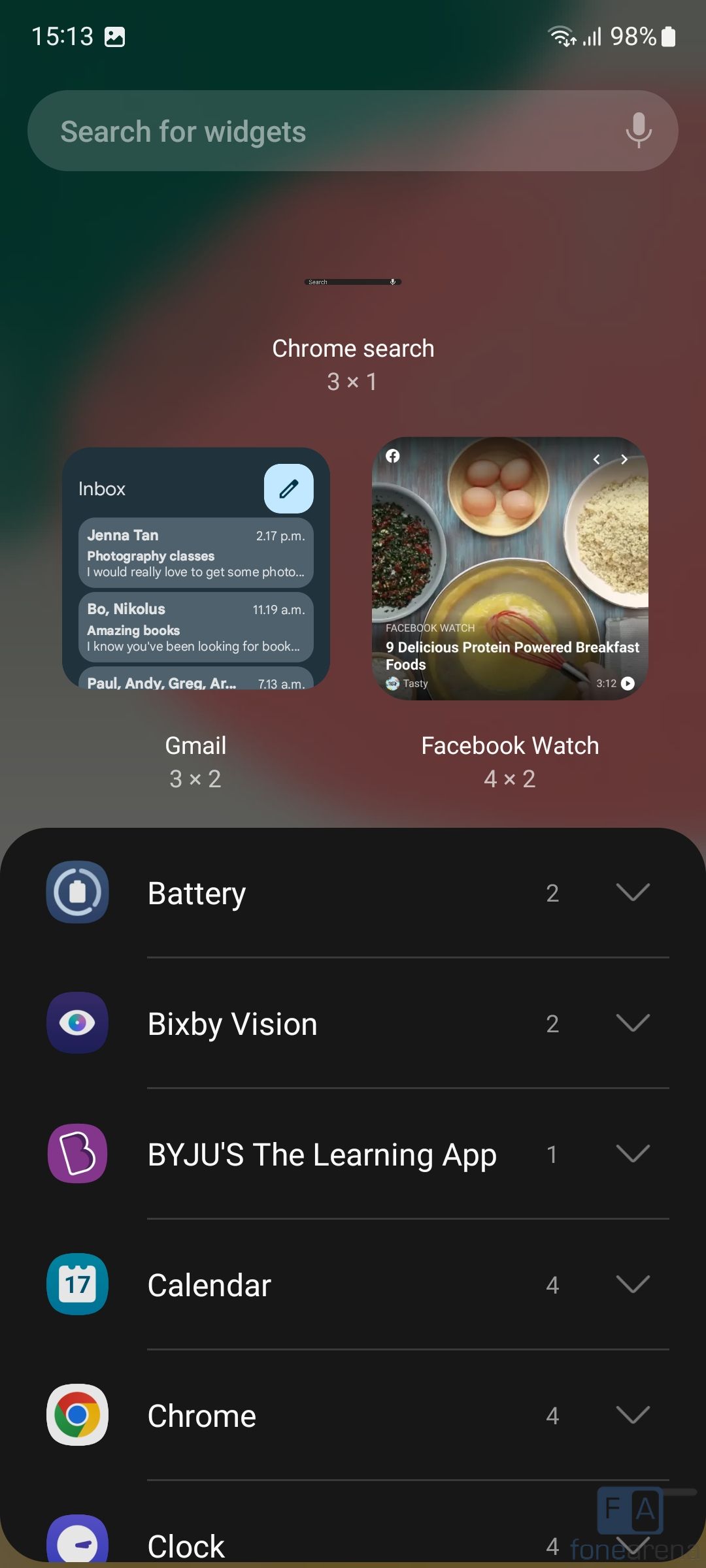This vertical rectangular image, presumably a screenshot from a smartphone, is rich with details. In the upper left corner, the current time is displayed in white font, while the upper right corner shows the battery status, also in white. The very top of the image features a black background, transitioning into a reddish-brown or brown hue on the right side.

At the very top, spanning horizontally from left to right, is a search box. Centered at the top of the page within the search box, the words "Chrome Search" are displayed in white font, accompanied by "number three times, and then it's one."

Below the search box, the screen is divided into two vertical rectangular sections. The first section on the left is predominantly black with the word "Inbox" in white font. In the upper right corner of this section, there is a white square icon depicting a pen. Below this, there are several unreadable entries, except for the top one, which appears to be a name—James Tan—with three entries listed, though the third is partially cut off. Under these entries, the text "Gmail" appears, followed by "three times two."

The vertical section adjacent to it on the right displays an overhead view of four brown eggs in a bowl. To the right of the bowl is a light-colored bowl filled with rice. At the bottom, there is another bowl, possibly containing egg yolk or a mix of eggs, with a mixer beside it. There is also an unclear object to the left. Beneath this image, in white font, partially obscured, the text reads "protein powdered breakfast foods."

Further down, in white font once again, it states "Facebook watch four times two."

The bottom part of the screen reverts to a black background with white text, featuring icons and words in bold font. From left to right, these include:
- "Battery" with a number "2" and a downward-pointing arrow beside it.
- "Bixby Vision," also with a number "2" and a downward arrow.
- "By J-U'S," followed by "the learning app" with a number "1" and another downward arrow.
- "Calendar" accompanied by the number "4" and a downward arrow.
- "Chrome" with a downward arrow.
- "Clock" also with a downward arrow.

Each word is prefaced by a corresponding icon.